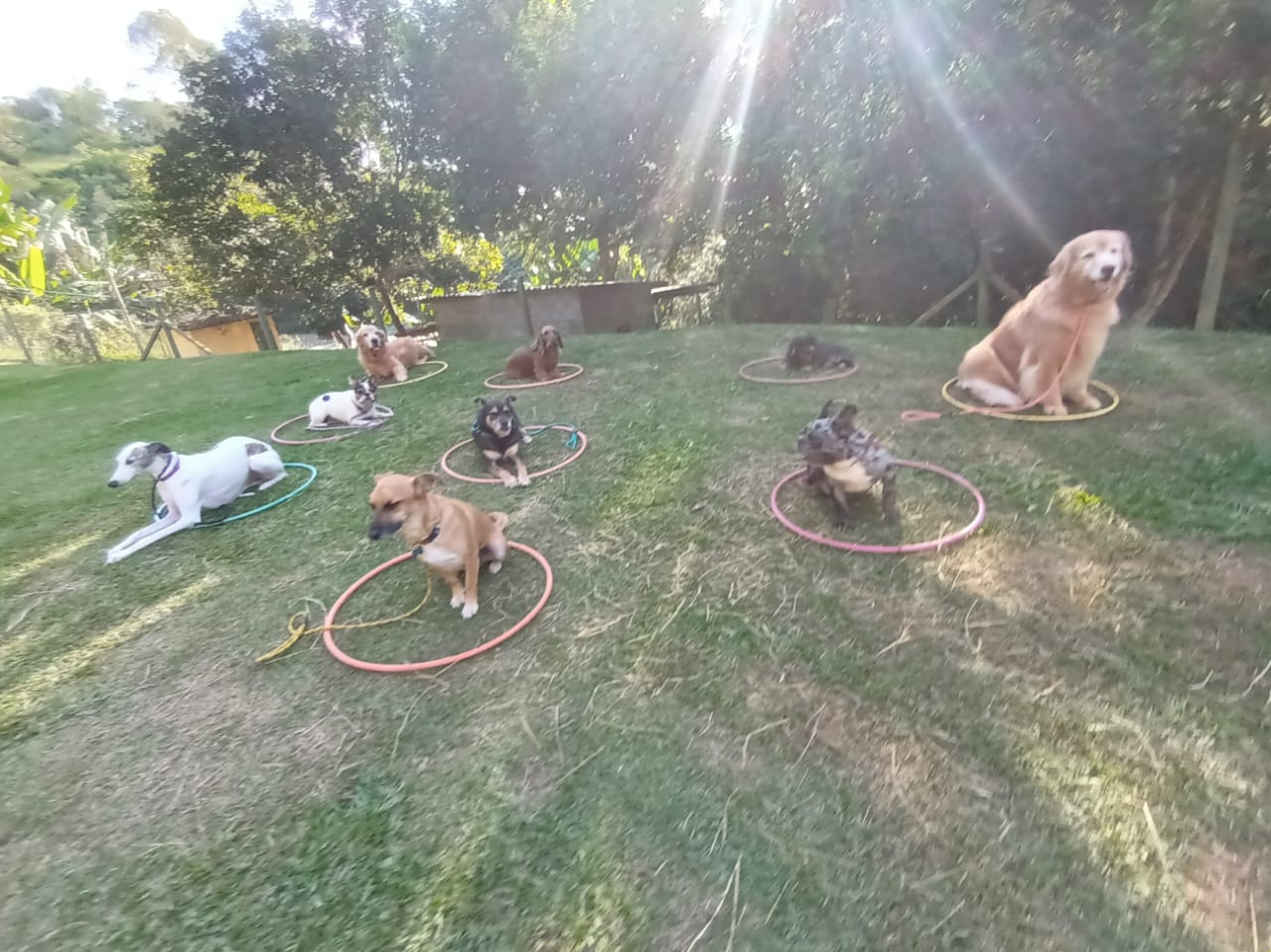The photograph captures an outdoor scene with a diverse assembly of dogs, each sitting inside brightly colored hula hoops positioned on a grassy field. The sun illuminates the scene, casting warm rays from the top right, with additional sunlight filtering through a dense row of verdant trees in the background. The field of grass in the foreground shows patches where the grass is matted and slightly dead.

The dogs are arranged in vertical rows. On the left, a trio of dogs includes a brown Collie, a white Bulldog, and a white Greyhound, all facing forward. Behind them, in another row, is a brown Cocker Spaniel, a black Terrier, and another brown dog, giving the impression of attentive poise. Toward the right, there are two more dogs aligned vertically: a Cocker Spaniel lying down and a Bulldog sitting upright. In the upper right corner, a lone Collie sits attentively in his hoop.

Distinctively, there are two golden retrievers: one positioned on the far right, and another lying down further back to the left. The other dogs vary in size and breed, including a mix that resembles French Bulldogs, a Basset Hound with long ears, and a small black and tan dog. Behind the dogs on the left, there is a hint of fencing and wooden structures, adding depth and context to the scene. The backdrop is filled with lush, full trees of varying shades of green, enhancing the natural, serene setting. The hula hoops in pink, yellow, and green contribute a playful and orderly contrast to the natural environment.